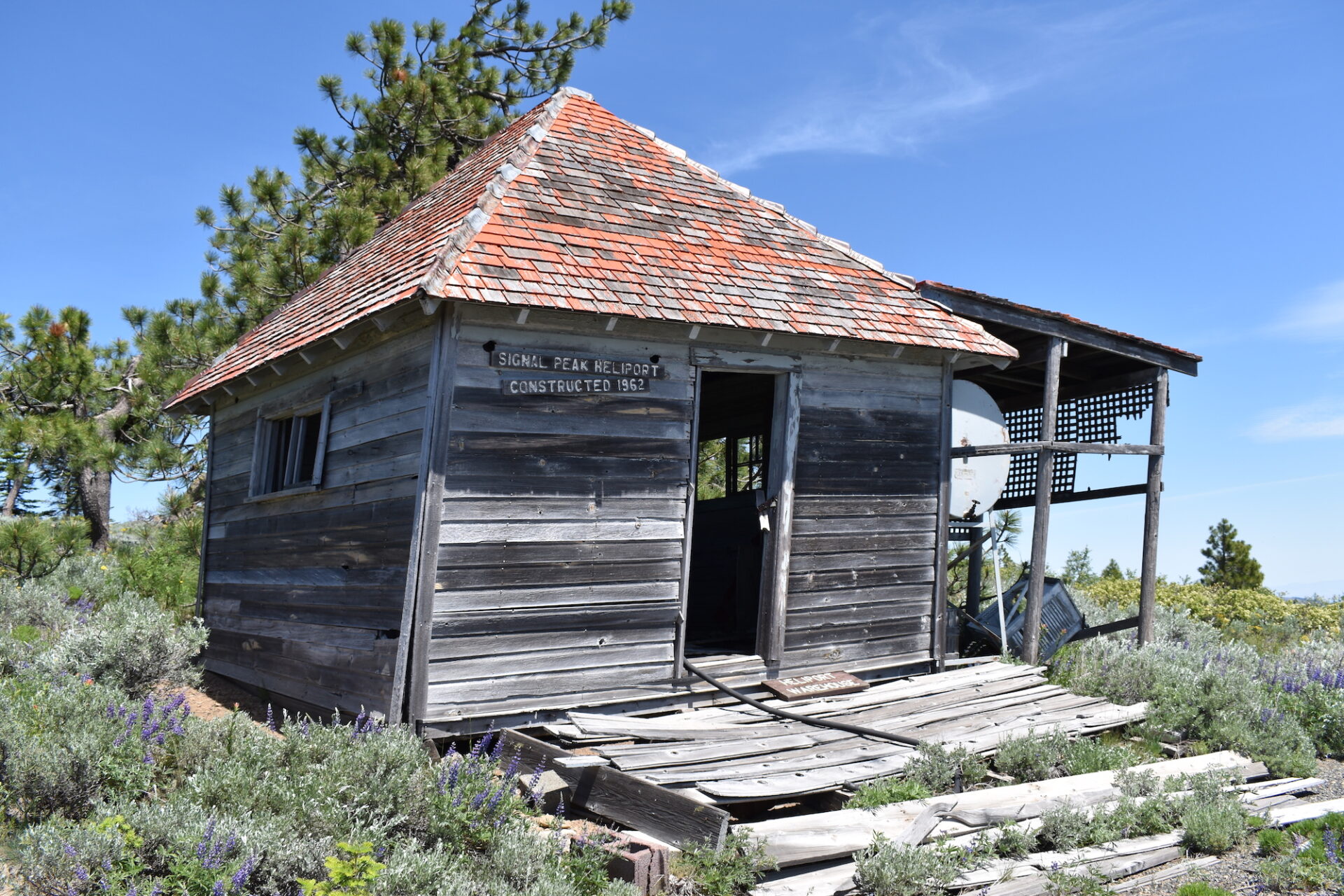The image captures a detailed view of a rustic, abandoned wooden shack labeled "Signal Peak Heliport, constructed in 1962," situated in a vibrant outdoor setting. The shack, featuring aged, darkened walls and a thatched brick roof, appears dilapidated and slightly tilted to the right, though its roof remains in relatively decent condition. Surrounding the shack is a hot and lush landscape with a mix of desert and forest elements, under a clear blue sky with minimal clouds. Flanking the scene on both sides are various trees, shrubs, and vibrant plants, particularly in shades of white and purple. A makeshift wooden walkway made of planks leads up to the entrance of the shack, adding to the rustic charm of the environment. In the foreground, there is an indecipherable sign on the ground, hinting at further history and mystery about the heliport.